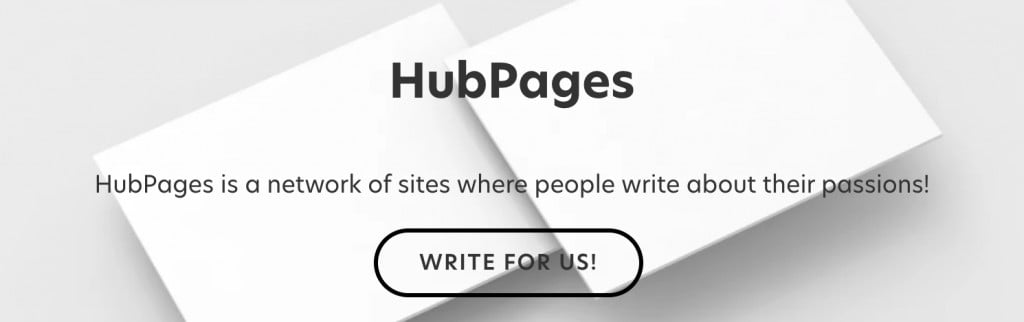This digital advertisement features a sleek, minimalist design with a significantly elongated rectangular shape, approximately following a 20:80 height-to-width ratio. The background is a light gray, almost white hue, likely derived from a stock photo. Superimposed over this backdrop are two slightly angled white rectangles, with the right rectangle overlapping and positioned slightly higher than the left, causing the top edge to be cut off by the image boundary and casting a subtle shadow.

Prominently displayed in the upper-central part of the image is bold black text reading "HubPages," with capitalized 'H' and 'P'. Directly beneath this title, smaller text explains, "HubPages is a network of sites where people write about their passions!" punctuated enthusiastically by an exclamation mark. At the bottom of the image, a prominent call-to-action button invites viewers with the message, "Write for us!"